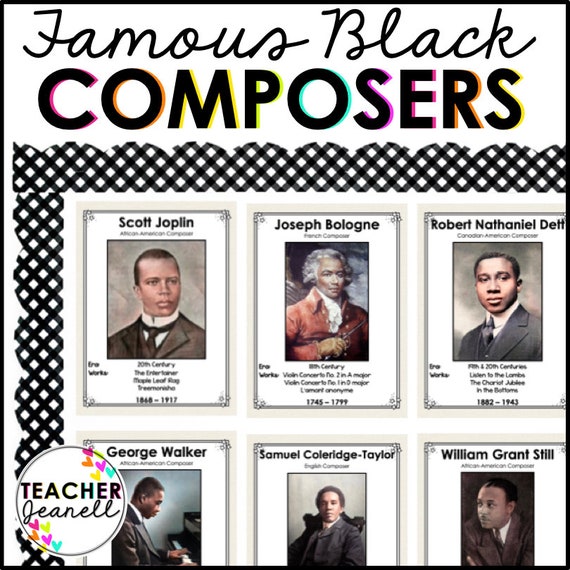This vibrant poster titled "Famous Black Composers" features an array of historical and influential black composers. The title is elegantly presented with "Famous Black" in black cursive font, while "Composers" is in bold, block letters highlighted in a rainbow gradient of red, orange, yellow, green, turquoise blue, pink, red, and yellow. The poster is bordered by a striking black and white crosshatch pattern. 

At the top left, the first flyer celebrates Scott Joplin. Next to Joplin is Joseph Ballone, and to his right is Robert Nathaniel—though unfortunately, part of his last name is cut off. Below, starting on the far left, the next flyer honors George Walker. The middle flyer is dedicated to Samuel Coleridge-Taylor, and the final flyer on this row highlights William Grant Still.

Inset pictures of each composer accompany their names, along with their birth and death dates, although the latter information is partially obscured in the bottom row. In the left corner, a circle reads "Teacher Janelle," adding a personal touch to this educational collage.